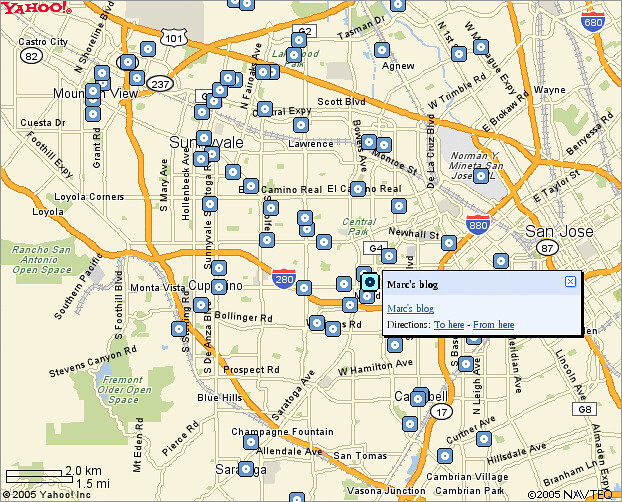This image is a screenshot of an online map from Yahoo, as indicated by the red "Yahoo" logo in the upper left-hand corner. The map depicts the city of San Jose, California. Prominent roads are highlighted in yellow, such as Route 280 running east-west, Route 880 running north-south, and other thoroughfares including Route 101 and Route 87. Railroad tracks stretching east-west are also visible towards the top. The map's background is rendered in beige.

At the center of the map, there is a blue rectangle labeled "Marks Blog," repeated directly below along with interactive options for directions to and from this point. Scattered throughout the map are small blue squares with a white circle or the letter 'O' inside, whose specific purpose is unclear but may be related to "Marks Blog."